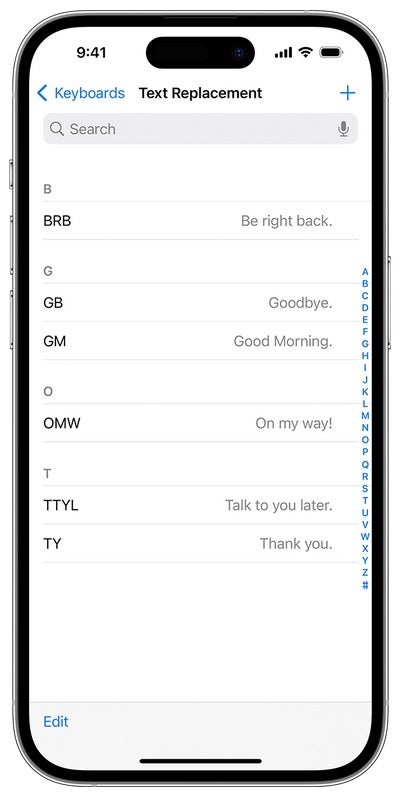A smartphone is depicted in the image, encased in a sleek silver case. The phone features three silver buttons on the left side and one on the right. Highlighting its edges, a black outline frames the screen. At the top of the phone, a small black oval houses a camera lens on the right side. The time on the phone is displayed as "9:41" in black text.

The status bar at the top shows strong reception with four black bars and a fully lit black Wi-Fi icon, indicating a robust internet connection. The battery icon indicates that the phone is fully charged.

On the screen, the "Text Replacement" settings page is open. A blue-highlighted heading on the left reads "Keyboard," beneath which "Text Replacement" appears in black. Adjacent to this, a blue "+" icon is displayed. Below this are several gray rectangles and icons, including a search bar with a gray magnifying glass and microphone icon.

The screen displays various text replacement shortcuts, each listed with a black abbreviation on the left and its corresponding expanded phrase in gray on the right:
- "BRB" (Be right back)
- "GB" (Goodbye)
- "GM" (Good morning)
- "OMW" (On my way!)
- "TTYL" (Talk to you later)
- "TY" (Thank you)

Each phrase is separated by a line. At the bottom-right corner of the screen, the word "Edit" is prominently displayed in blue with a capital "E."